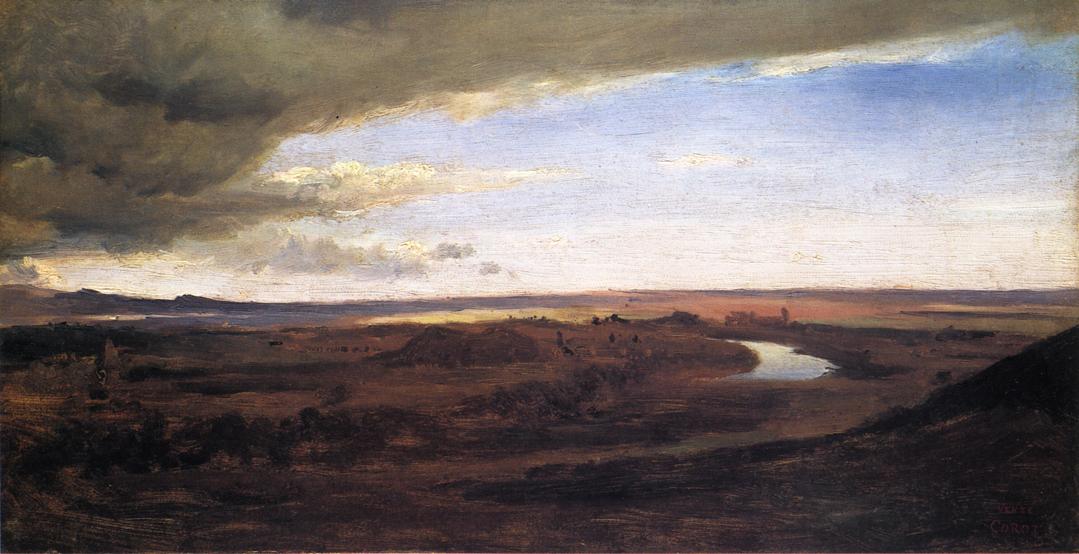This painting captures a somber landscape dominated by a small, winding river set amidst a predominantly brown terrain, evoking a clay-like texture. The river, although partially visible, forms a subtle curve through the flat expanse. Rolling hills, or perhaps low foothills, provide a modest backdrop, their muted presence reinforcing the subdued palette of the scene. The sky overhead is tumultuous, heavily clouded on the left and center, hinting at an impending storm, with dark gray and black clouds obscuring a portion of the underlying blue sky. The right side of the sky shows a slight easing of cloud cover. The overall tone is dark and earthy, suggesting an evening or dusk setting. Despite the intricate details of water and sky, the landscape mostly remains a blend of brown and dark hues, with no vivid greens or lively elements. Scattered dots and specks, possibly trees or distant wildlife, punctuate the otherwise still, desolate scenery. The painting lacks clear brush strokes, leaning more on the overall impression to convey the meditative and stark beauty of this natural vista.